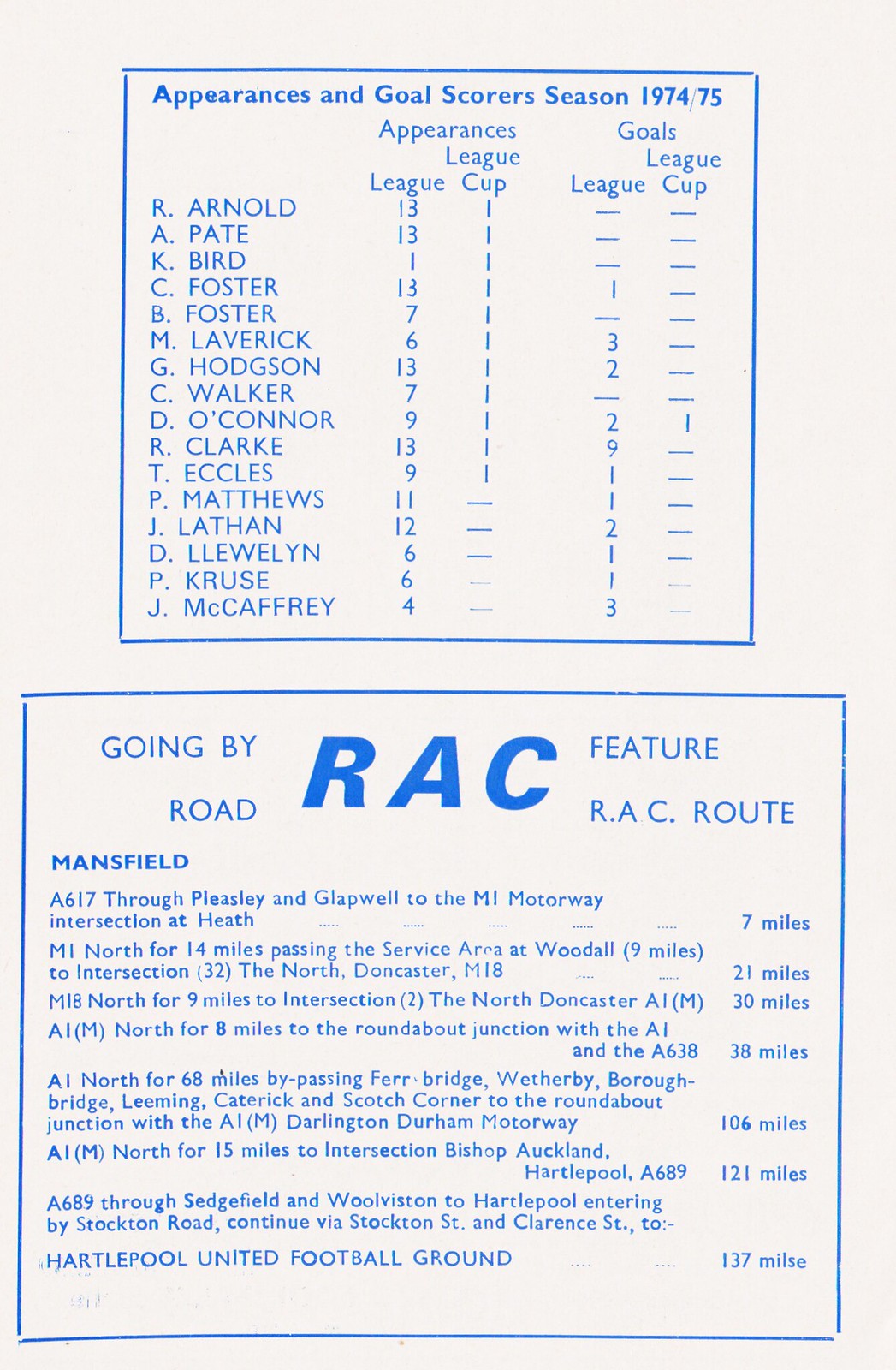This image depicts a page from a Game Day program or magazine, showcasing a clean white background with all text and borders meticulously printed in blue ink. The page is divided into two distinct sections. The top section, bordered in blue, is titled "Appearances and Goal Scorers Season 1974-75". It features a detailed list of around 15 players, including their names, the leagues they participated in, their appearances, and goal statistics for both the league and cup competitions during the 1974-75 soccer season.

Below this, the lower section is titled "Going by Road Feature, RAC Route" and prominently displays the acronym "RAC" in bold blue letters. This section provides detailed directions and distances for traveling to Hartlepool United Football Ground, mentioning specific routes such as the A617 through Pleasley and Glapwell to the M1 motorway intersection at Heath. The left column of the section includes the directions while the right column lists the distances, indicating this part appears to be related to road travel information.